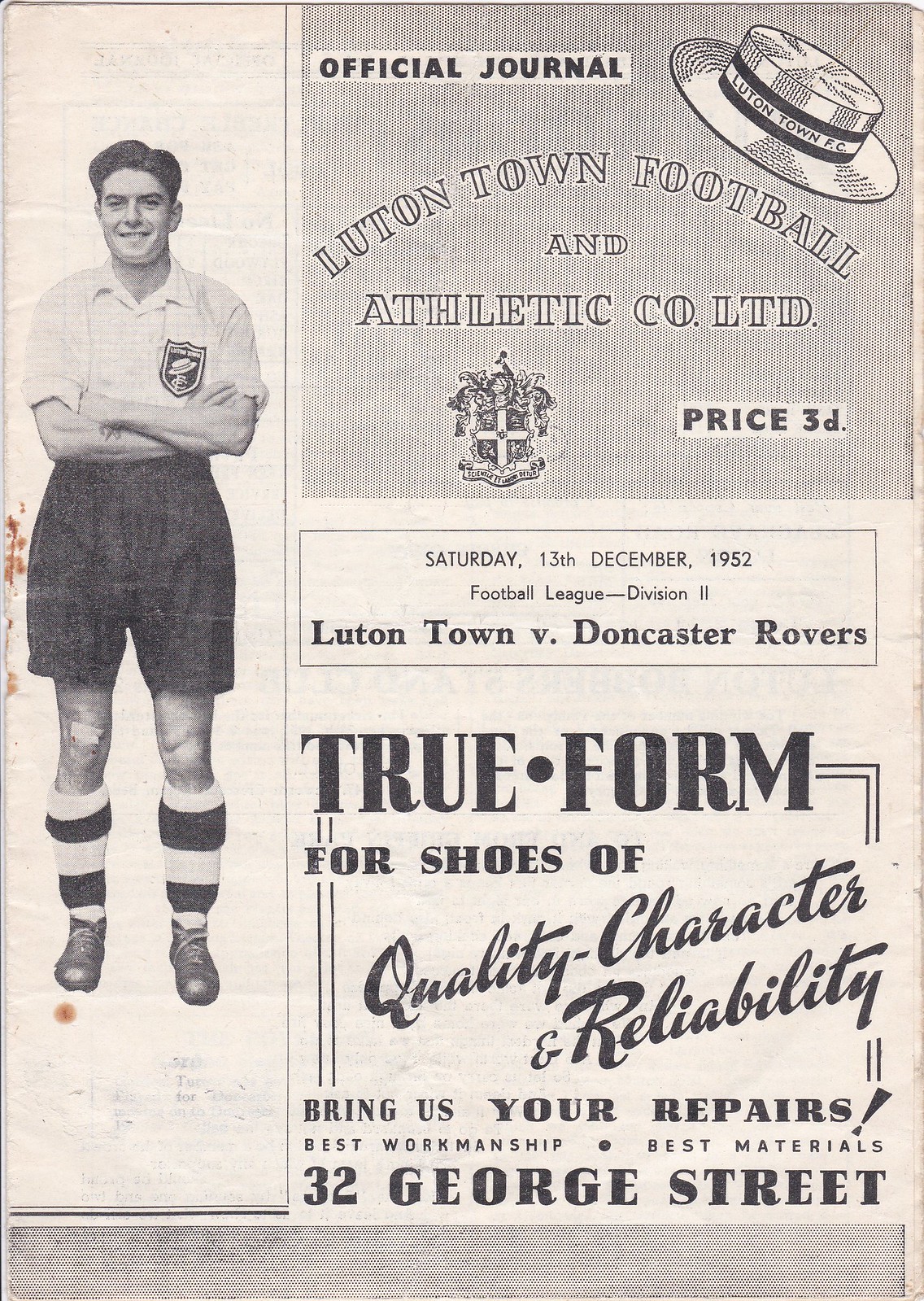This is an image of an old, black-and-white promotional flyer that appears slightly pink in hue. At the top, bold black text reads "Official Journal," and just below it, "Luton Town Football and Athletic Company Ltd." is prominently displayed. The flyer features an image of a smiling British football player wearing a white shirt with a shield that says "Luton Town," dark pants, and white-and-dark socks, along with shoes. 

Additionally, there is a hat and an emblem, possibly of the Luton Town football team, with "Price 3D" noted nearby. Below the main heading, it announces a Football League Division II match: "Luton Town vs Doncaster Rovers," scheduled for Saturday, 13th December 1952. 

In the lower right corner, there's an advertisement for a shoe store emphasizing "True Form for Shoes of Quality, Character, and Reliability" with a call to "Bring Us Your Repairs," promising the "Best Workmanship, Best Materials." The store's address, "32 George Street," is also included.